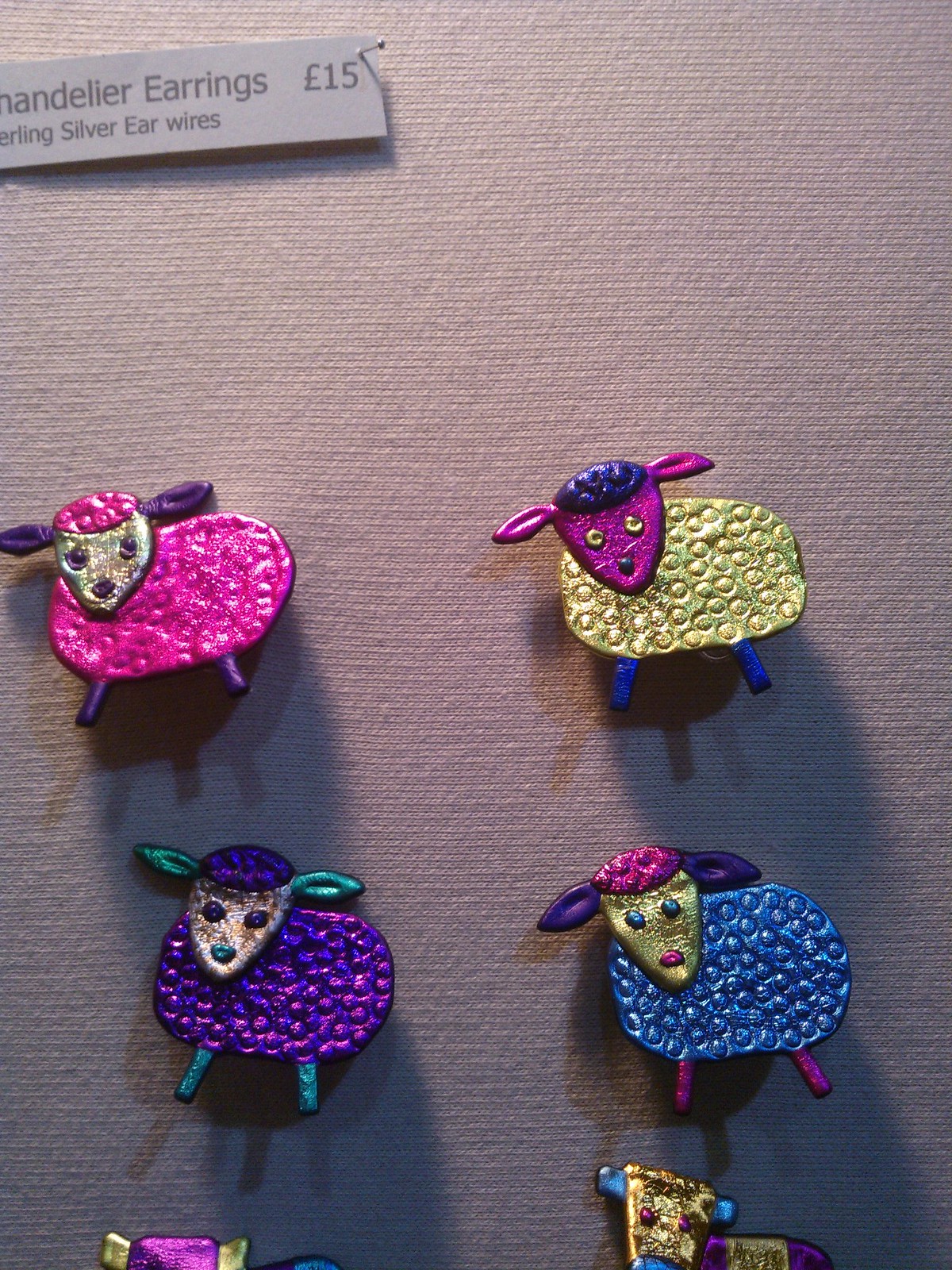This image showcases a collection of brightly colored, handmade earrings and brooches shaped like animals. The display features six decorations arranged on a textured, fabric-covered board that appears to be either light gray or pinkish. In the upper left corner, there's a partially visible label that reads, "chandelier earrings, 15 pounds, sterling silver ear wires," though the first few letters are cut off.

At the top, four decorations form a square, representing lambs. Each lamb is uniquely colored:
1. The upper left lamb has pink wool, a yellow face, and purple ears, eyes, nose, and legs.
2. The upper right lamb features a white body, purple wool on its head, a pink face and ears, yellow eyes, a black nose, and blue legs.
3. The left middle lamb has purple wool, a golden face, turquoise ears and nose, purple eyes, and green or turquoise legs.
4. The right middle lamb shows off blue body wool, pink head wool, a gold face, purple ears, blue eyes, a pink nose, and pink legs.

Below the lambs, two cow-like creatures are partially visible:
1. The left one displays yellow horns, a pink head, and a hint of a blue back.
2. The right one has a gold head, blue horns and nose, red or purple eyes, and a purple body with a yellow middle part.

These intricate pieces appear to be handcrafted from clay, exhibiting a metallic finish and a variety of vibrant colors, adding a playful, artistic touch to the collection.